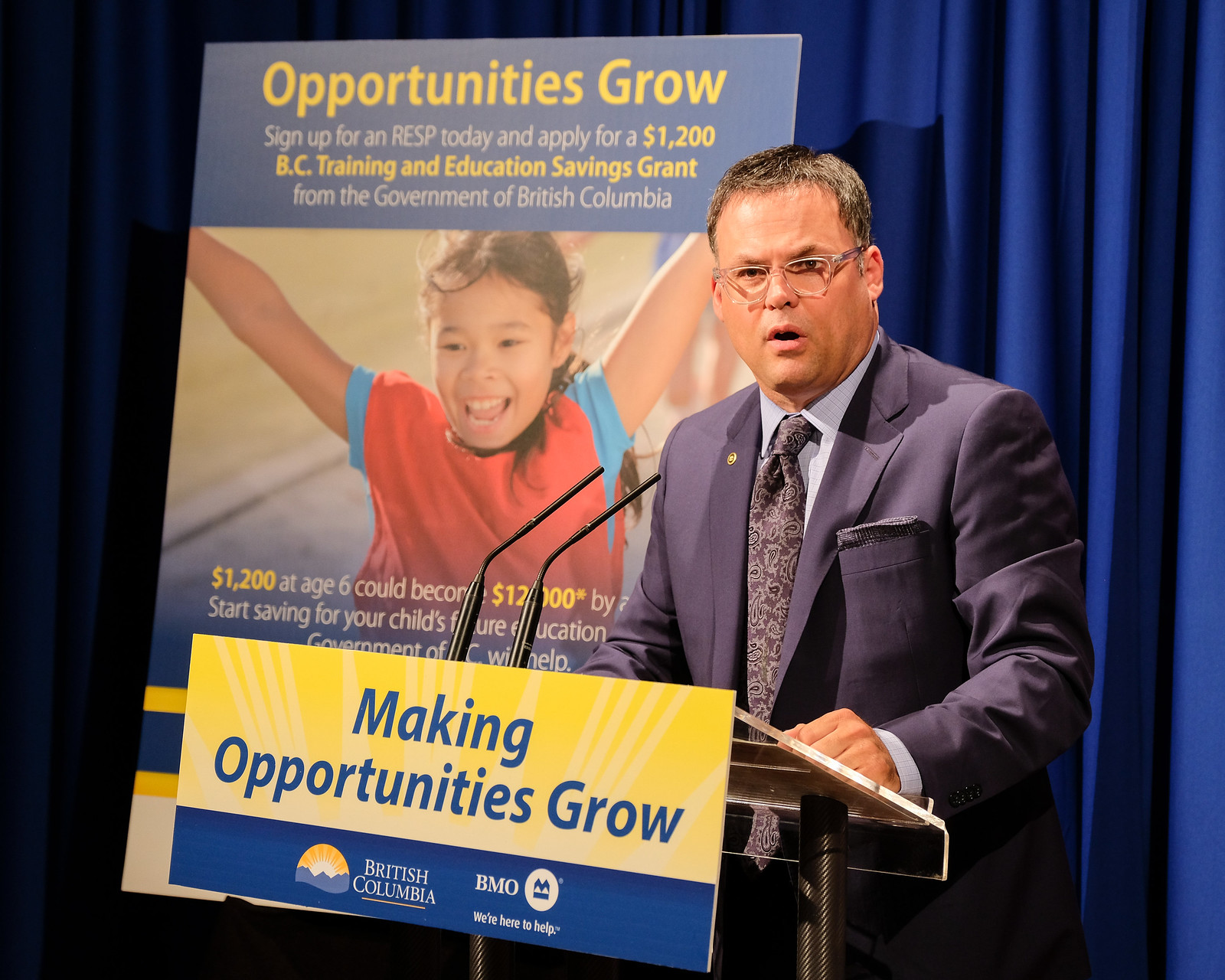In this detailed and vibrant photograph, we see a man standing behind a glass and metal podium, giving a presentation. He is dressed in a dark bluish-gray suit with a light blue button-up shirt underneath, complemented by a plum-colored paisley tie and a matching handkerchief peeking out of his suit pocket. The man has short hair and wears glasses, with a pin on his lapel and a pen in his pocket. His hands rest firmly on the podium as he speaks into two microphones, his mouth open mid-speech.

The podium features a prominent blue and yellow sign displaying the words "Making Opportunities Grow, British Columbia, BMO. We are here to help." In the background, a thick blue curtain stretches across the scene, creating a formal backdrop. Slightly to the left behind the man, there's a large banner with gold and white text against a blue background. It promotes a financial grant with the message: "Opportunities Grow. Sign up for a RESP today and apply for a $1,200 B.C. Training and Education Savings Grant from the Government of British Columbia." The banner also depicts a young girl joyfully raising her arms, capturing attention and adding a touch of warmth to the formal setting. This well-composed image captures a moment of public speaking, layered with context and visual details.